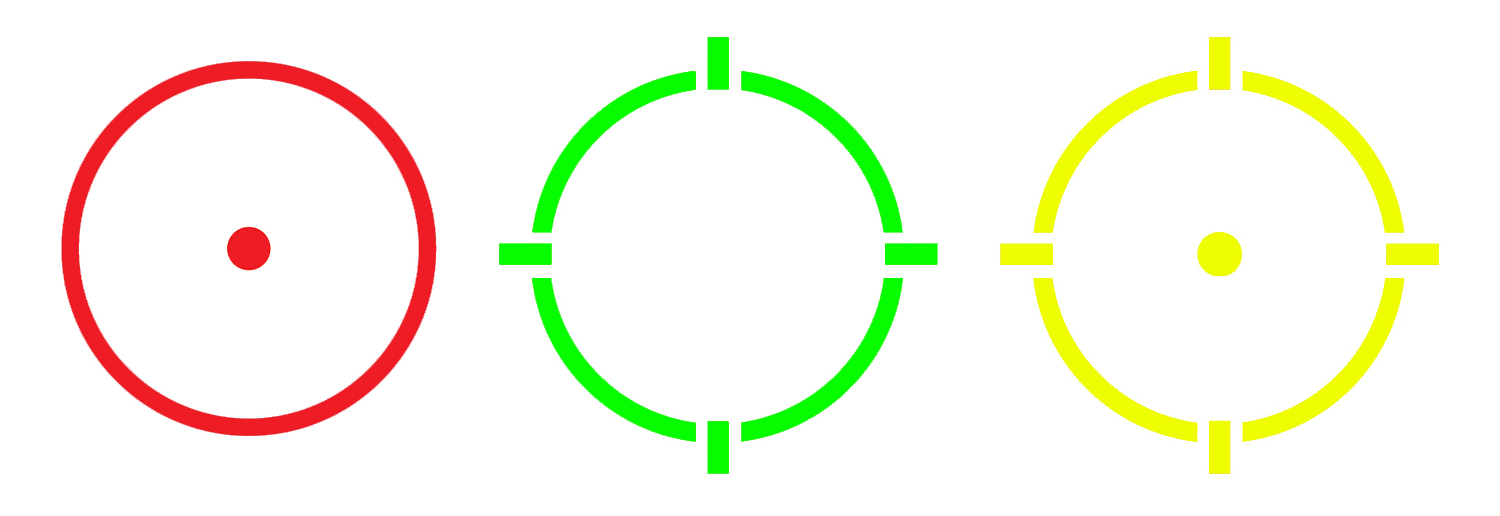The image features three distinct circles arranged horizontally against a plain white background. Starting from the left, the first circle is solid red with a uniform red dot in its center. The middle circle is light green with a unique design, featuring lines that divide the circle at the cardinal points—top, bottom, left, and right. The last circle on the right is yellow and combines elements from the other two; it has a yellow dot in its center and yellow lines segmenting the circle in the same cardinal directions. The background is uniformly white, offering a stark contrast that highlights the details within each circle.